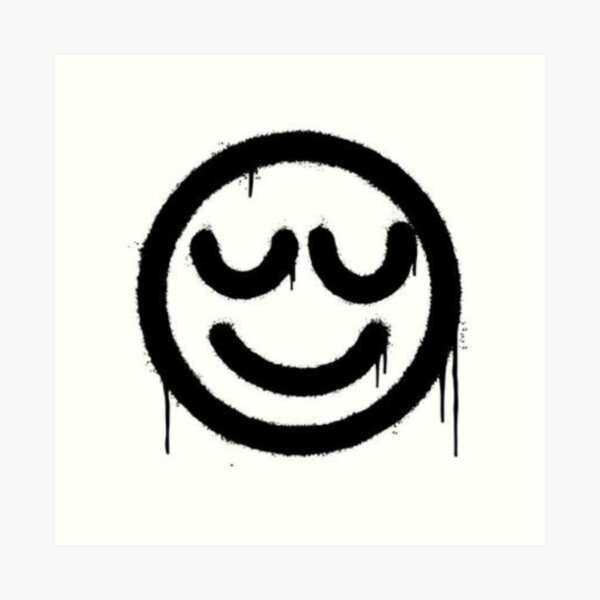The image is a square artwork measuring approximately four inches by four inches, bordered by a pale bluish-gray half-inch frame. Inside this frame lies a white background with a subtle pinkish hue. At the very center, a black spray-painted circle, about an inch and a half in diameter, prominently features a simplistic smiley face. The eyes of the smiley are shaped like small, lowercase "u"s, from whose outer right corners black paint drips down. Similarly, drips also emanate from the right side of the smile. Additional drips of black paint extend from the circle: two on the right-hand side, one on the upper left, and another on the lower left. The overall aesthetic of the image is defined by its spray-painted style, with the drips enhancing the raw, unfinished look of the art. The image contains no text, focusing purely on the visual elements of the smiley face against the lightly tinted white background, framed thoughtfully by its bluish-gray border.